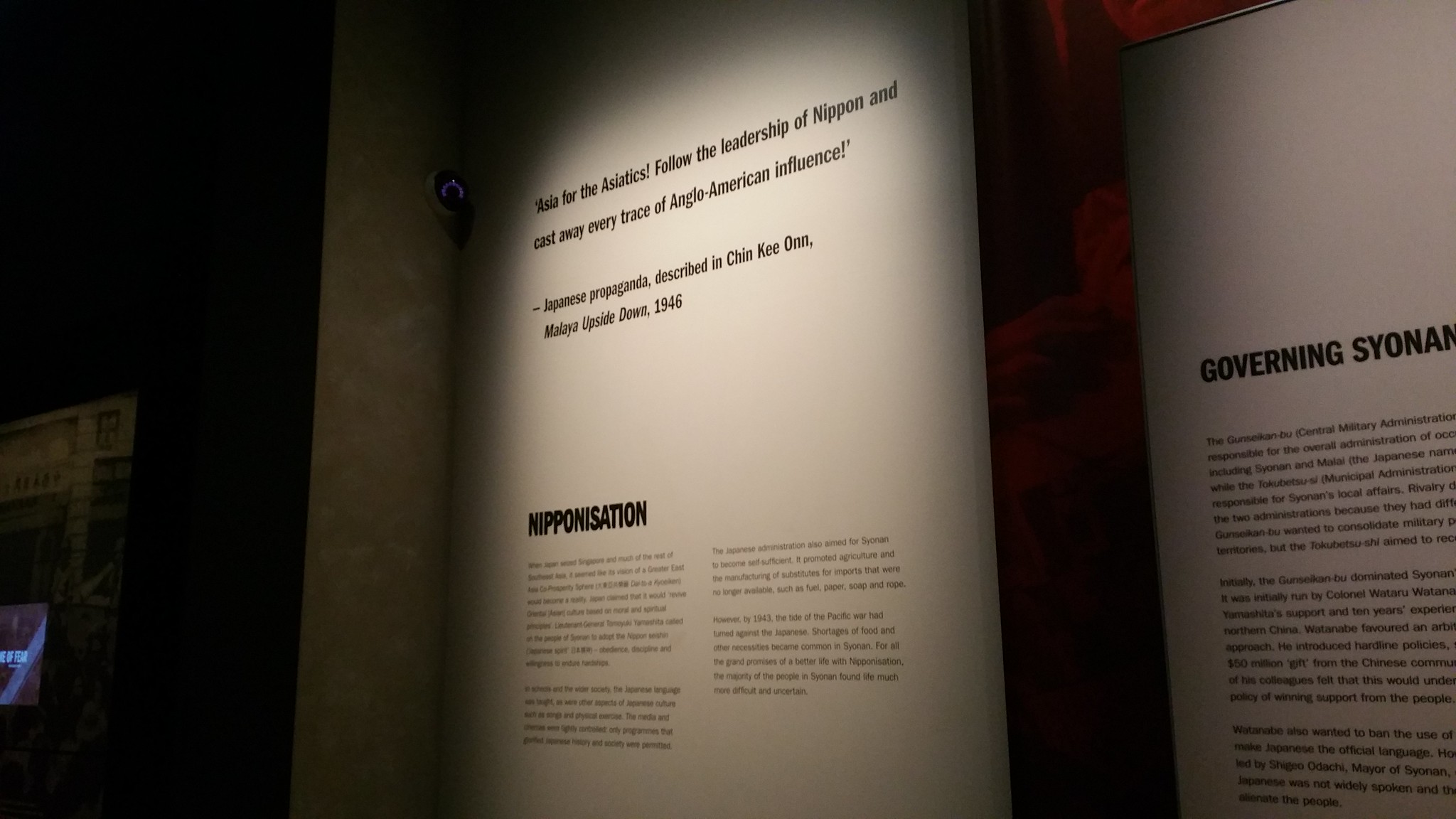This image appears to be of a museum exhibit wall, divided into three distinct sections. The left third of the image is a dark black strip, with a faint hint of white along its edge, though it's difficult to discern what this white area contains. The central section features a white background illuminated by a light, with prominent black text that reads, "Asia for the Asiatics, follow the leadership of Nippon and cast away every trace of Anglo-American influence." This is identified as Japanese propaganda described in Chin-Chi-On, Maya upside down, 1946. Below this, there is more white space followed by the bold word "Nipponization," beneath which are two columns of small, difficult-to-read text in black font, arranged over four paragraphs. 

The right third mirrors the central section with a similar white background and small black text. It contains the title "Governing Sionan," although this text is cut off in the image, followed by another segment of black font text that is equally challenging to read due to its size. The overall setup suggests that this is part of a museum exhibit, with the text describing historical Japanese propaganda efforts, all displayed on walls under focused lighting in a dimly lit room.